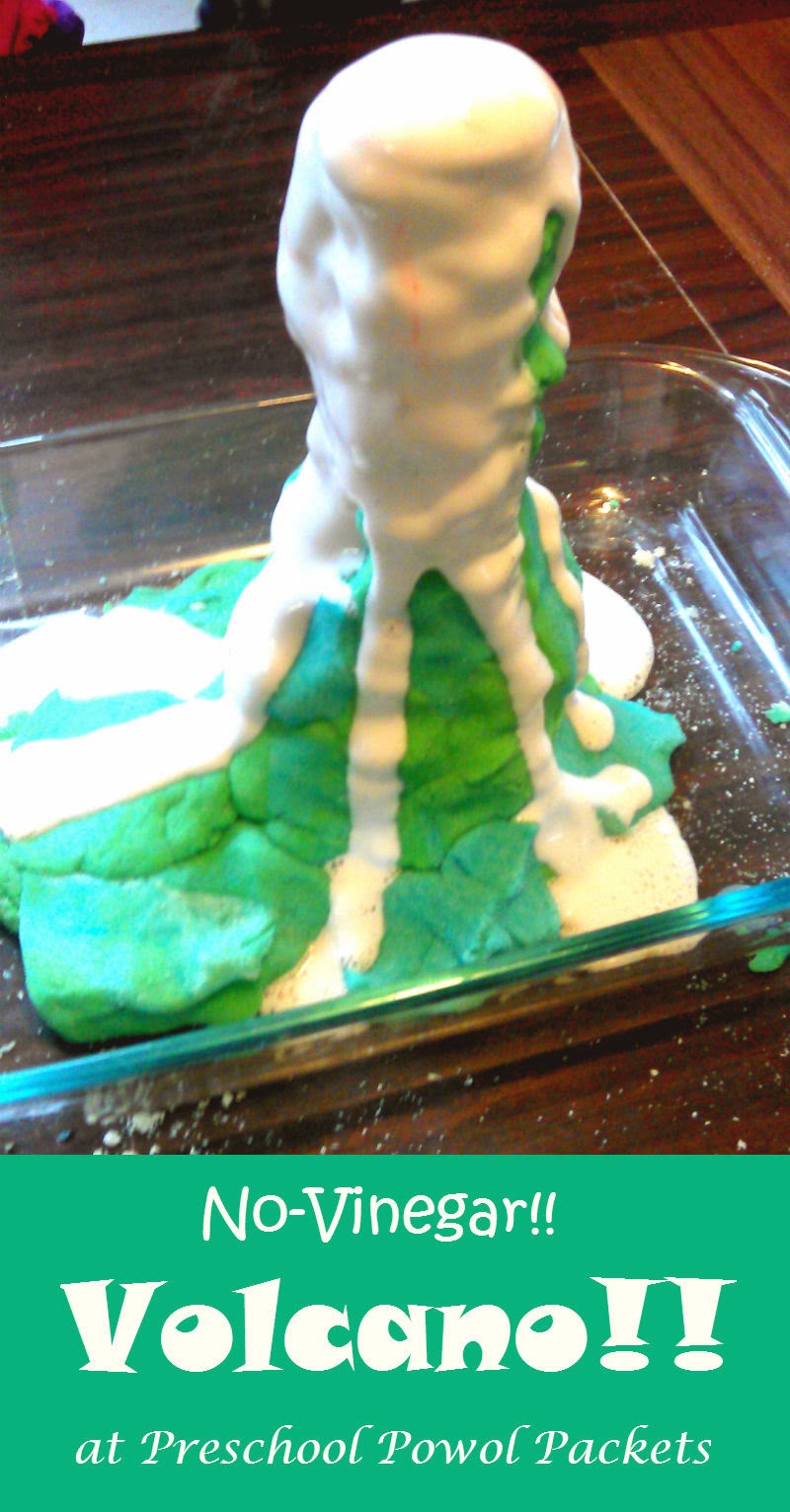The image depicts a detailed and colorful school project showcasing a volcano model. The volcano itself is primarily green at the base, transitioning into white at the top, where a foamy substance appears to ooze down its sides, mimicking lava. This creatively crafted volcano is positioned within a glass roasting pan, which stands on a wooden floor or table. Key textual elements in the image include a bold exclamation reading, "No vinegar!!" followed by "Volcano" and additional text indicating it is part of a preschool project associated with "Powell packets." The volcano's structure is either made from materials resembling Play-Doh or clay, or possibly an edible treat like melted marshmallow icing draped over a cake, suggesting it could be a fun, hands-on educational activity for young children.